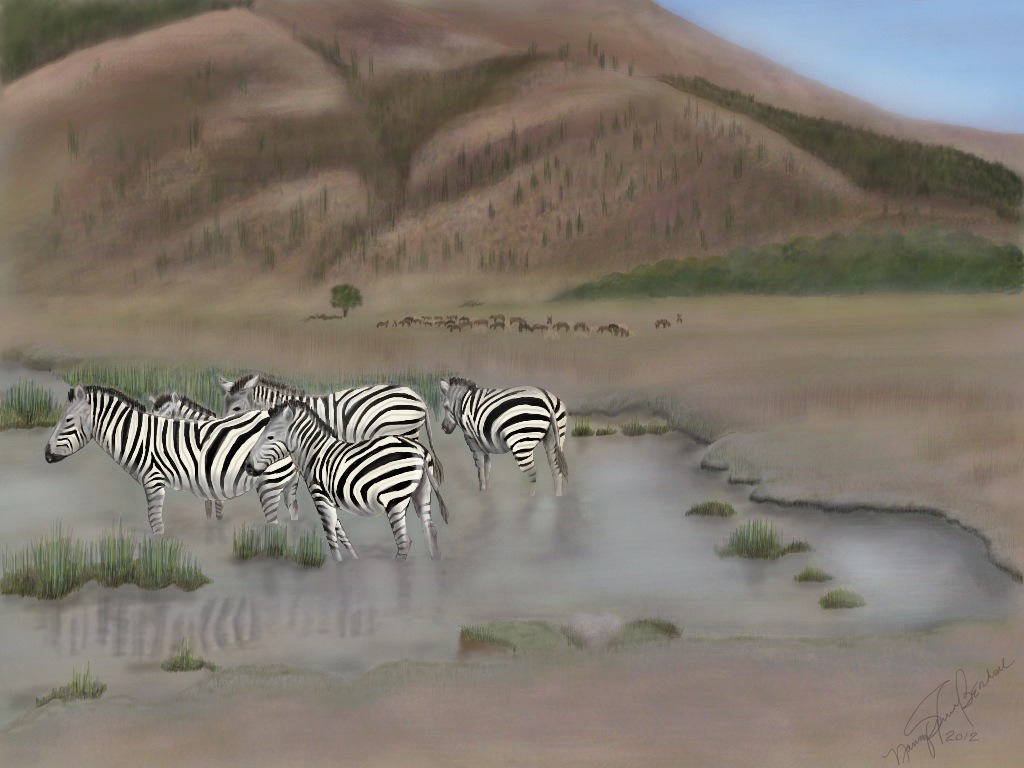The image is a detailed digital painting, blending elements of illustration and photography, depicting a serene African landscape. Central to the composition, five adult zebras with characteristic black and white stripes and a black mane stand in a shallow watering hole. The water is clear enough to see some sprigs of grass and a few lily pads, and it reflects the zebras' striking patterns. Surrounding the watering hole is a broad, muddy plain of varying brown shades, indicative of a dry season.

In the background, a series of hills and mountains stretch across the horizon, painted in earthy tones of tan, brown, and cream. Scattered across these mountains are sparse green trees and patches of vegetation, with a particularly prominent cluster of greenery to the right. The terrain transitions smoothly from the plains to the more rugged, soft-focus mountains, highlighting the expansive African landscape.

Dotted throughout the distant plain are small, brownish animals, possibly buffalo or hyenas, roaming freely. A solitary tree stands out amidst these animals, adding to the sense of isolation and vastness of the scene. Above, a clear blue sky frames the entire composition, completing the tranquil and natural setting.

The painting is signed by the artist in brown cursive in the lower right corner, dated 2012, adding a personal touch to this vivid portrayal of wildlife and nature.